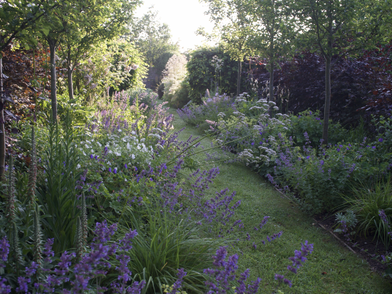The photograph captures a vibrant and well-maintained garden stretching approximately 50 yards, bathed in daylight. A diagonal green lawn path runs through the center, seemingly leading to a stone at the back. Flanking this path are diverse plants, including beautiful purple flowers, possibly lupines or purple bonnets, and striking white and yellow blossoms that could be goldenrod. On the left side, small cacti peek through amidst more clearly visible flowers. Bushes and low shrubs with off-white flowers populate the right side, bordered by lush, leafy trees. The background features a tall hedge and a tree adorned with white blossoms. The overall scene is lush and verdant, with sunlit patches indicating a bright, albeit slightly overcast day.